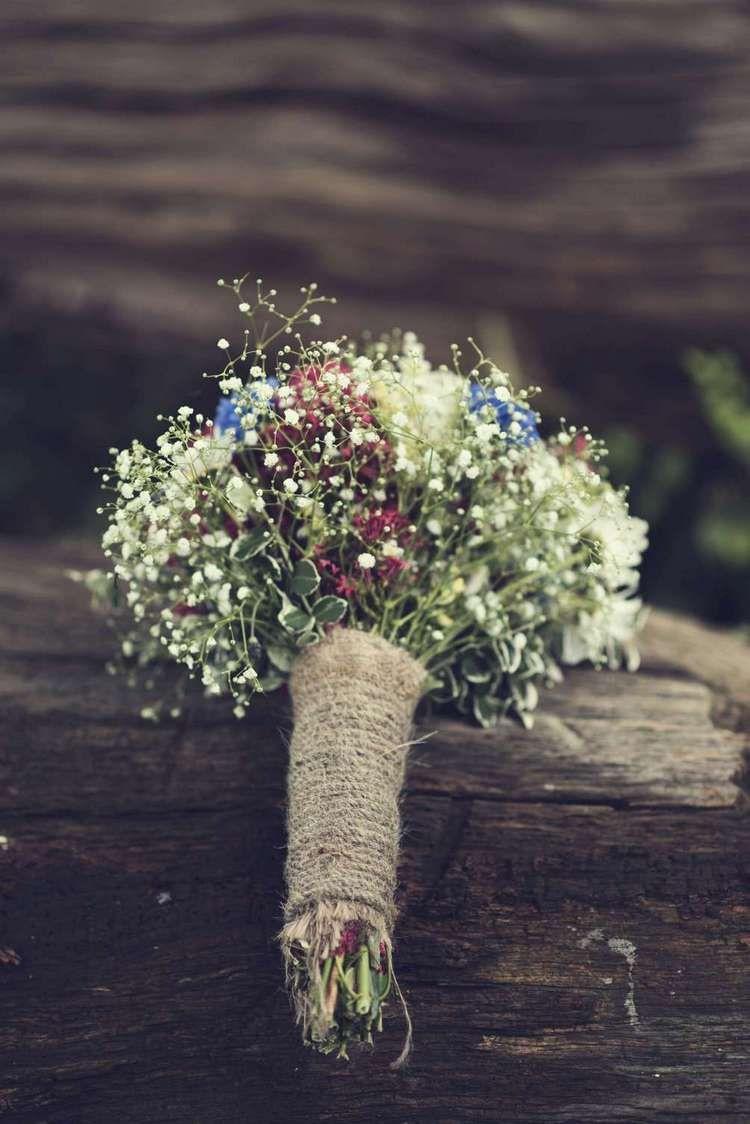This high-quality photograph captures a small bouquet of flowers, elegantly tied together with brown twine. The bouquet features an array of colors at the top, showcasing delicate white, blue, and purple flowers, along with hints of red mini flowers, with a predominant presence of baby's breath. The stems, which are thin, firm, and light green, are cut to varying lengths and extend out from the binding. The bouquet rests on a dark brown wooden platform, while the background remains artfully blurred, ensuring the focus stays solely on the floral arrangement. The overall composition and detail suggest a scene reminiscent of a wedding bouquet.